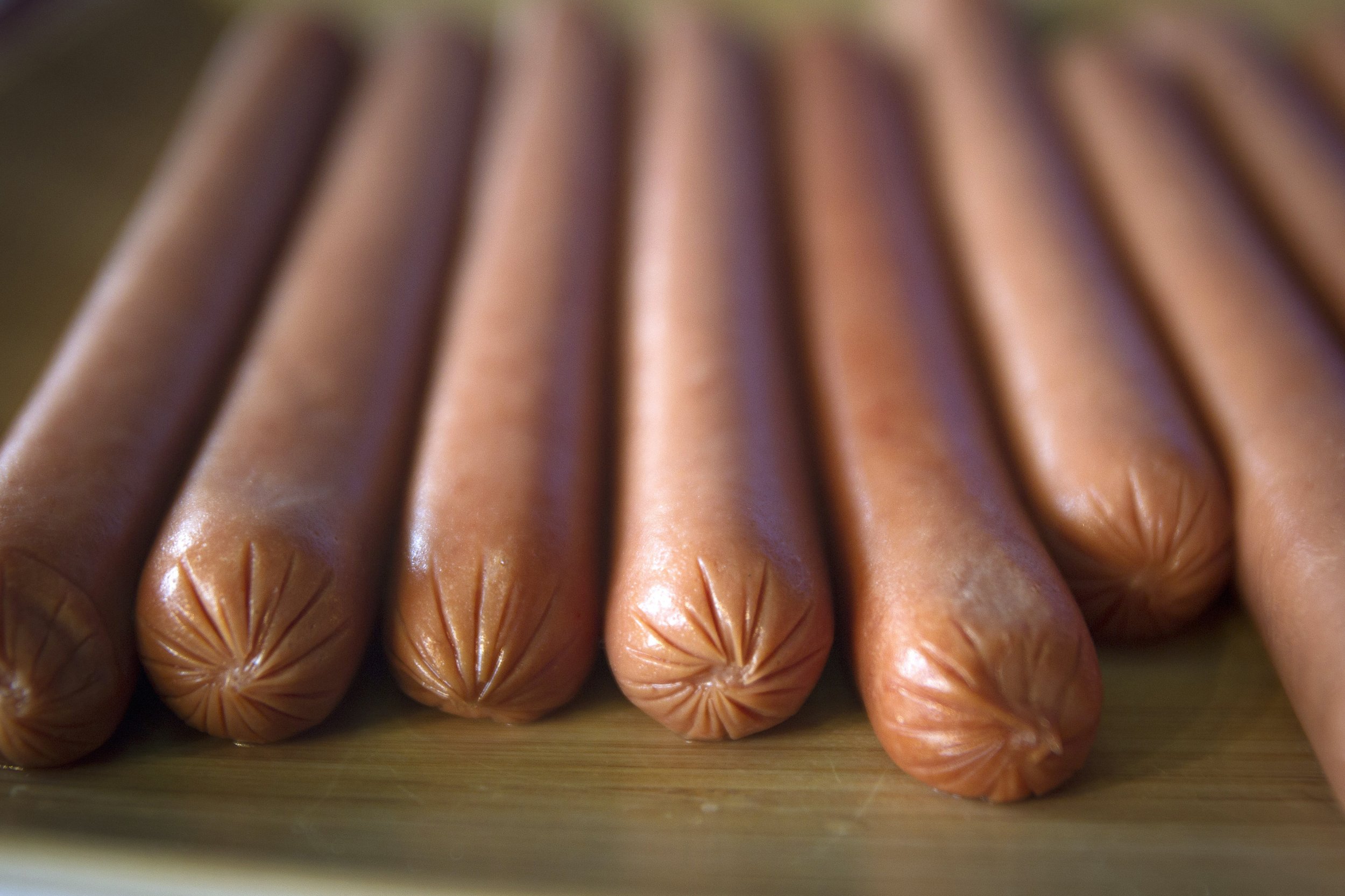On a rustic wooden table, there is a display of approximately 9 to 10 hot dog wieners. The wieners, which appear to be uncooked or possibly pre-cooked, are uniformly aligned and ready either for grilling or immediate consumption. Their distinctive brownish color and the characteristic bunched-up tops—formed by twisting the casing—confirm their identity as hot dogs. There are no grill marks on any of the sausages, implying they have not been grilled yet. The simplicity of the scene, with no other items in the background, places full emphasis on the presentation of the hot dog wieners.